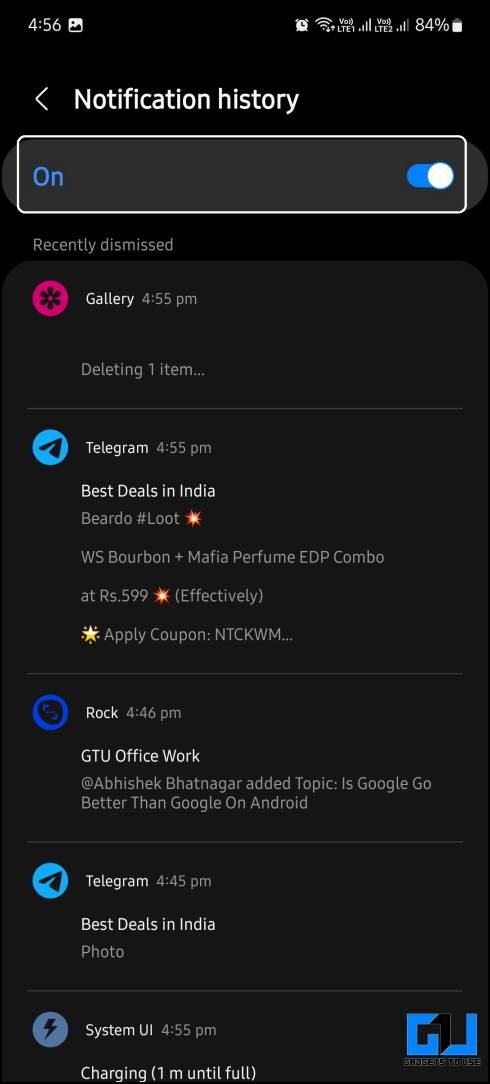The image captured from a cell phone screen displays the Notification History page set against a black background. At the top center of the screen, encased in a white-bordered box, the word "On" is highlighted in blue, indicating the active status of the notification history. To the right, a toggle slider is visible with a white circle positioned to the right, with the background of the slider shaded in blue, confirming that the feature is enabled.

Beneath this section, the "Recently dismissed" notifications are listed. The first entry shows an alert from the Gallery at 4:55 PM, indicating "Deleting one item." Next to the Gallery icon, there is a black flower symbol enclosed within a bright pink circle. Below this is a notification from Telegram, also at 4:55 PM, which reads "Best deals in India, Bernardo #loot." The Telegram icon features a white paper airplane inside a teal circle. Further down the list, notifications include "Rock" at 4:46 PM, another Telegram alert at 4:45 PM, and a System UI notification at 4:55 PM.